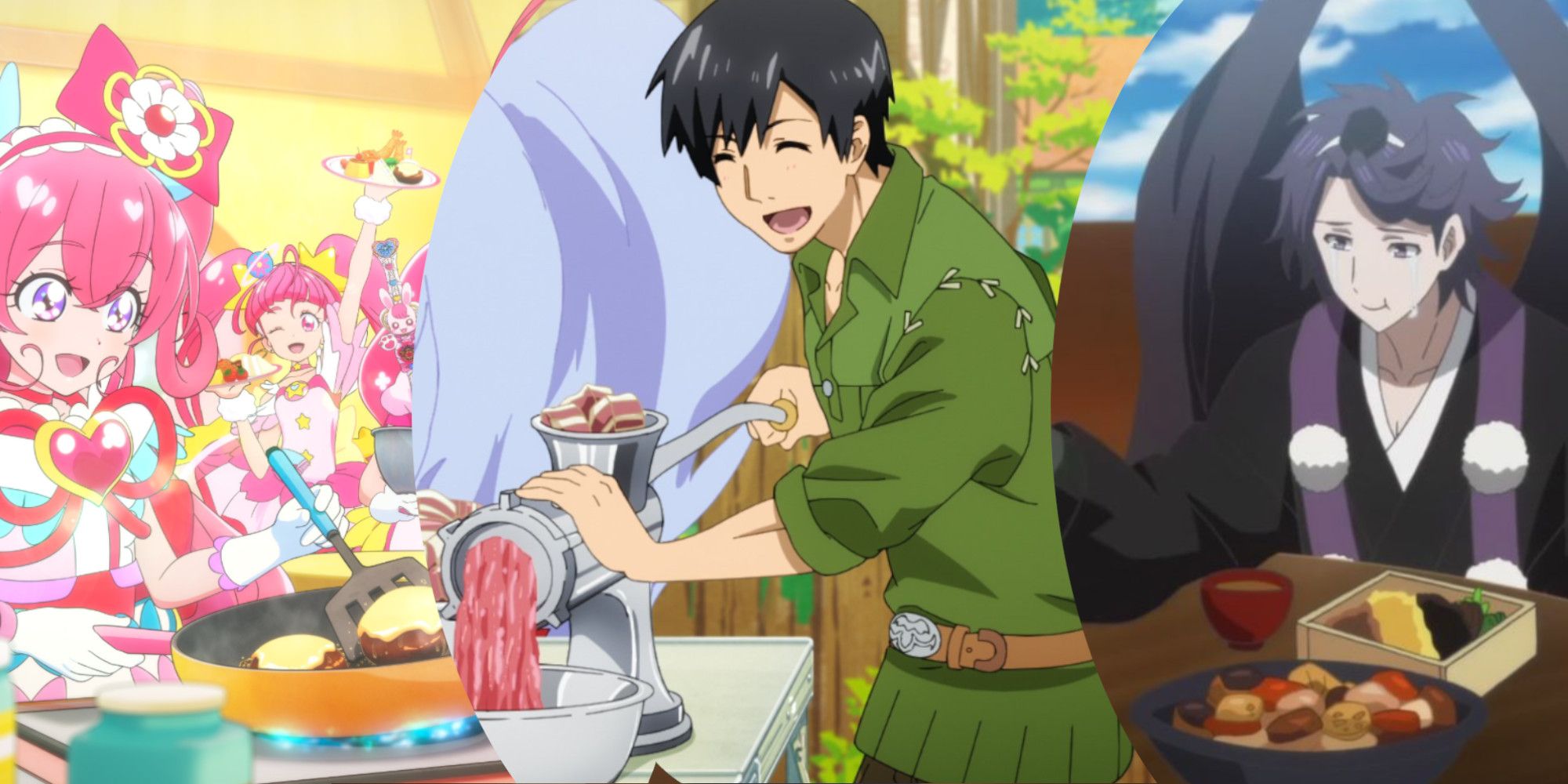This detailed Japanese animation illustration is divided into three parts, each highlighting distinct characters and scenes. On the far right, we see a light-complected woman with short, spiky, purple hair, sporting black wings, and wearing a long black robe with a purple, white-frilled scarf, and a white undershirt. She is seated at a brown table, visibly chewing with tears streaming down her face. In front of her, there is a light brown bento box containing neatly arranged yellow, black, and brown food with green garnish, a maroon bowl filled with a brown substance, and a pan featuring a mix of beige, red, light, and dark brown foods.

In the center, there is a young man with short black hair, dressed in a light green tunic with a light brown belt and a gray belt buckle. He operates a traditional silver meat grinder, turning pink and white meat into a fine maroon and pink paste that collects in a silver bowl beneath. The backdrop shows a wok on a stove cooking burger patties topped with white cheese, handled by a woman wielding a large spatula.

On the far left, multiple pink-haired girls with large pink bows adorned with flowers are depicted. They wear white and pink dresses with pink hearts and gold accents or pink bows at their necks. One girl is flipping cheeseburgers with a blue spatula in a mustard-colored pan, while another in the background raises two platters invisibly filled with various foods, such as shrimp, cheese, cherry tomatoes, and rice. Additionally, a cylindrical jar with a white lid is seen on the left side. The detailed artistry and vibrant color palette vividly bring the energy and diversity of the scenes to life.